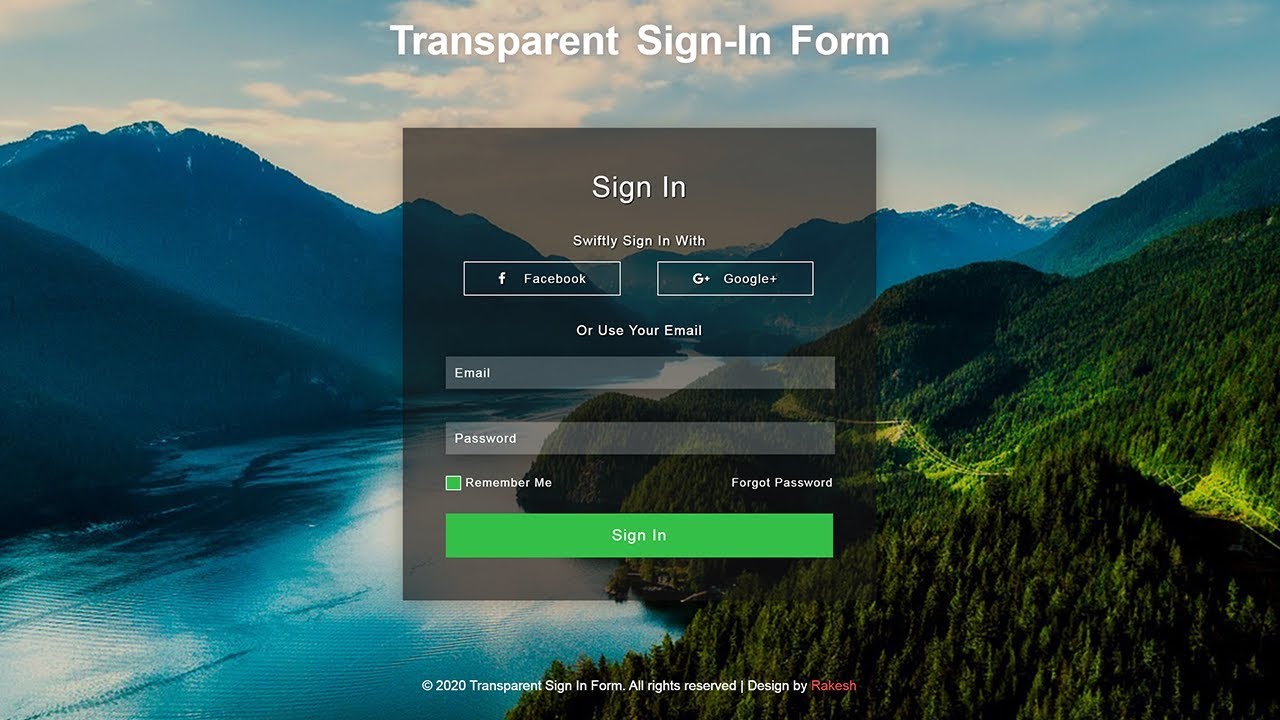The image features a partly cloudy sky over a majestic mountain range adorned with glaciers. Fog fills the valleys between the mountains, through which a winding river or lake can be seen snaking its way. Power lines cut through the dense forest at the base of the mountains, adding a touch of human presence to the natural scene.

Overlaying this picturesque landscape is a prominent, white, bold title at the top that reads "Transparent Sign-In Form." Beneath it, a grayed-out box instructs users to "Swiftly sign in with Facebook, Google, or use your email." Below this prompt, there are designated boxes for entering an email and password, accompanied by a "Remember Me" checkbox with a green highlight on the left. Additionally, there is a clickable "Forgot Password" link for users who need assistance. Further down, a green "Sign In" button stands out, inviting users to complete the sign-in process. At the very bottom of the overlay, it states, "Copyright 2020 Transparent Sign-In Form. All rights reserved. Designed by Rakesh."